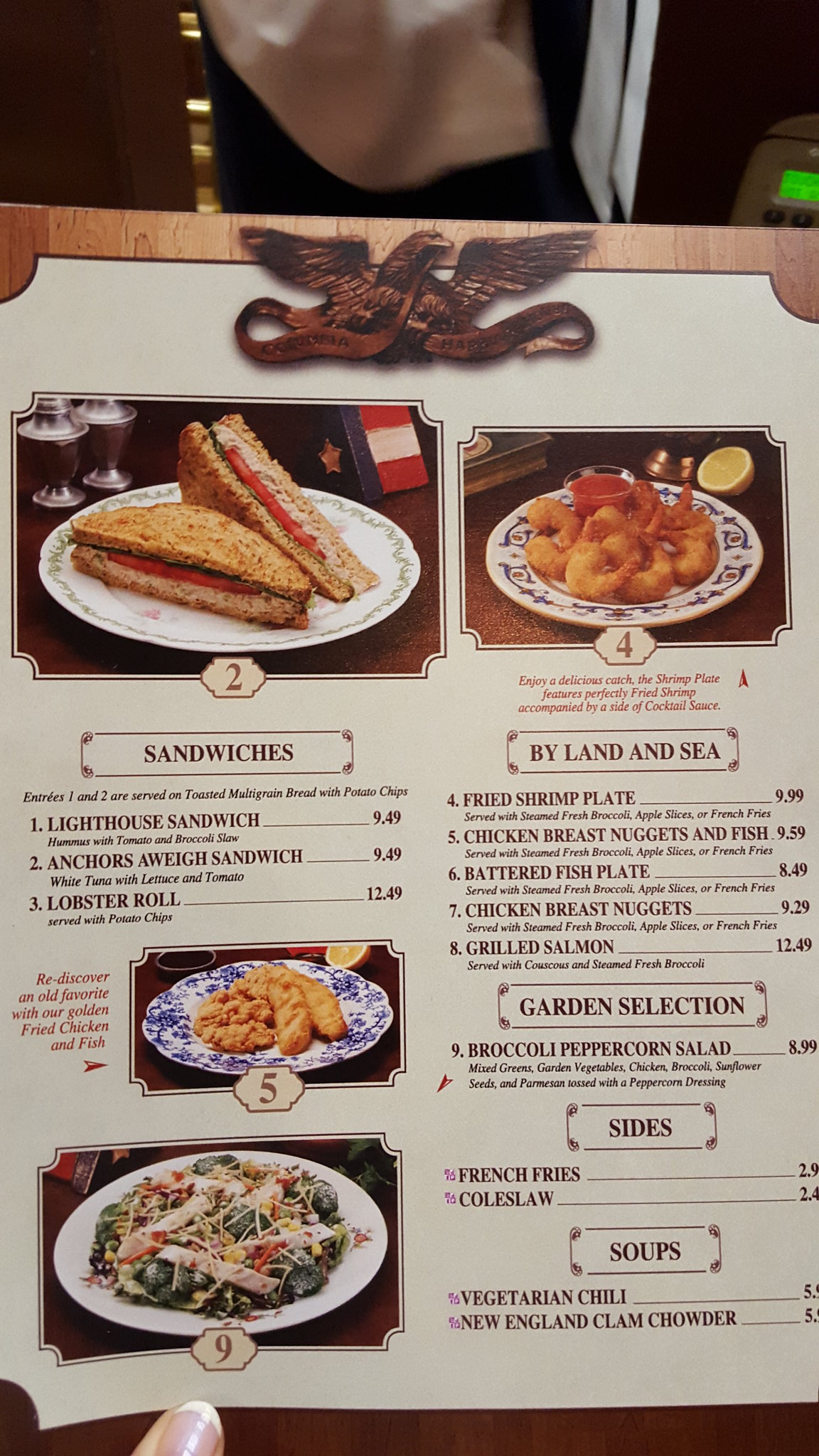The image displays a menu from a restaurant, showcasing a variety of food options. At the top of the menu, there is a logo resembling a statue of an eagle, accompanied by some text that is partially legible, including the word "Colombia" while the remaining words are unclear.

The menu features several photographs of dishes, each associated with a number for easy identification:
1. On the left, there is a picture of a sandwich labeled with the number 2, likely the "Anchors Away Sandwich."
2. On the right, a plate of shrimp is shown with the number 4, corresponding to the "Fried Shrimp Plate."
3. Another image features fried chicken with the number 5, indicating the "Chicken Breast Nuggets and Fish."
4. The final food photograph, labeled with the number 9, depicts a salad known as the "Broccoli Peppercorn Salad."

Additional menu items include a selection of sandwiches categorized as "by land and sea," a "Garden Selection" featuring the aforementioned salad, and sides such as french fries and coleslaw. The restaurant also offers a variety of soups, including vegetarian chili and New England clam chowder.